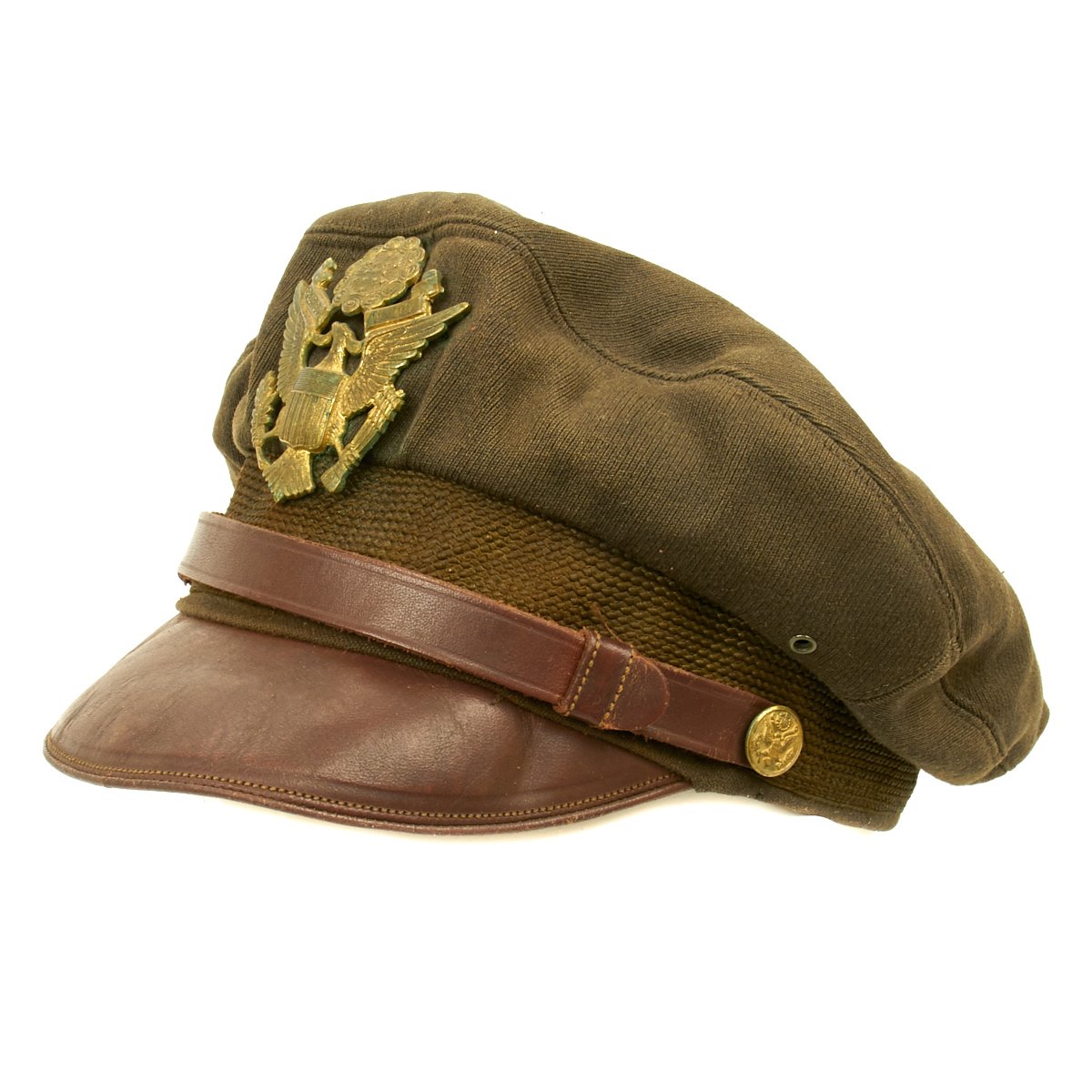The image showcases an old military hat, possibly from the World War II era, set against a stark white background. This vintage cap features a brown leather brim with detailed gold accents. Above the brim lies a textured, orangey-brown band resembling a canvas belt, secured by a gold button on the right side. A thinner burgundy stripe, made of the same leather material as the brim, overlays this band and also includes gold detailing. The top portion of the hat is a brownish-green canvas, slightly crumpled with a noticeable indentation at the very peak. Prominently displayed in the center is a large, elaborate gold emblem depicting an eagle clutching a shield and other elements in its talons. Another smaller gold circle with a similar emblem is located to the right of the main buckle. This meticulously detailed cap, likely worn by a cadet, presents a vivid historical artifact through its intricate design and craftsmanship.